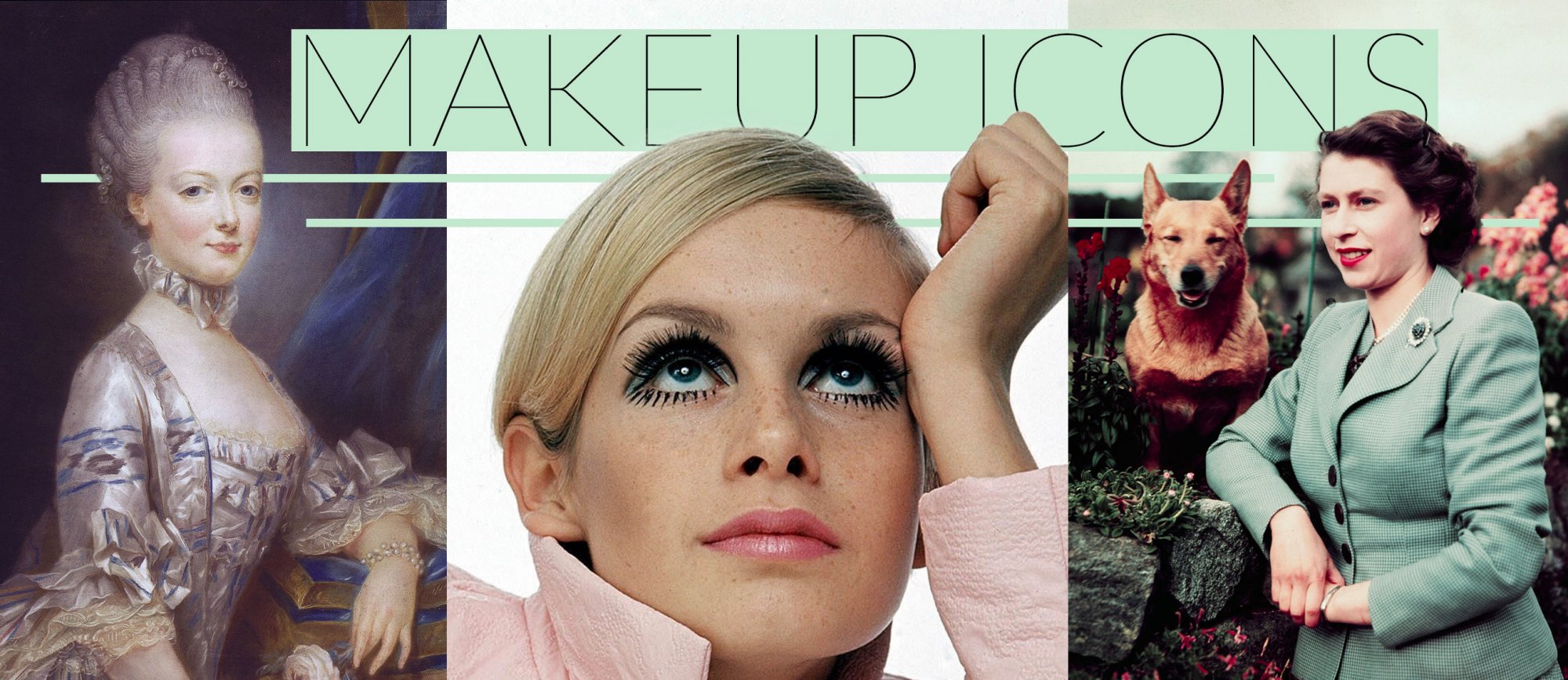This advertisement, set against a mint green background, features the words "Makeup Icons" in bold black text above three distinct images of women, each representing different eras and styles. 

To the far left, there is a painting of a possible French or English queen from the 1700s, reminiscent of Marie Antoinette. She is adorned in a powdered wig or an elaborate hairstyle typical of the period, and she wears a low-cut silver dress with blue and black prints, complemented by a choker.

The center image depicts a woman with an unmistakable 1980s vibe, possibly modeled after the iconic Twiggy. This photograph shows her with slicked and side-parted blonde hair, heavy eyeshadow, striking long eyelashes, and a light reddish-pink lipstick. She dons a pink jacket and gazes slightly upwards.

To the right, there is another contemporary woman who exudes a business-like demeanor. She is captured leaning against a wall in a garden, surrounded by flowers, with her happy expression accentuated by her green coat. Beside her stands a dog, potentially a corgi, adding a touch of warmth and companionship to the scene.